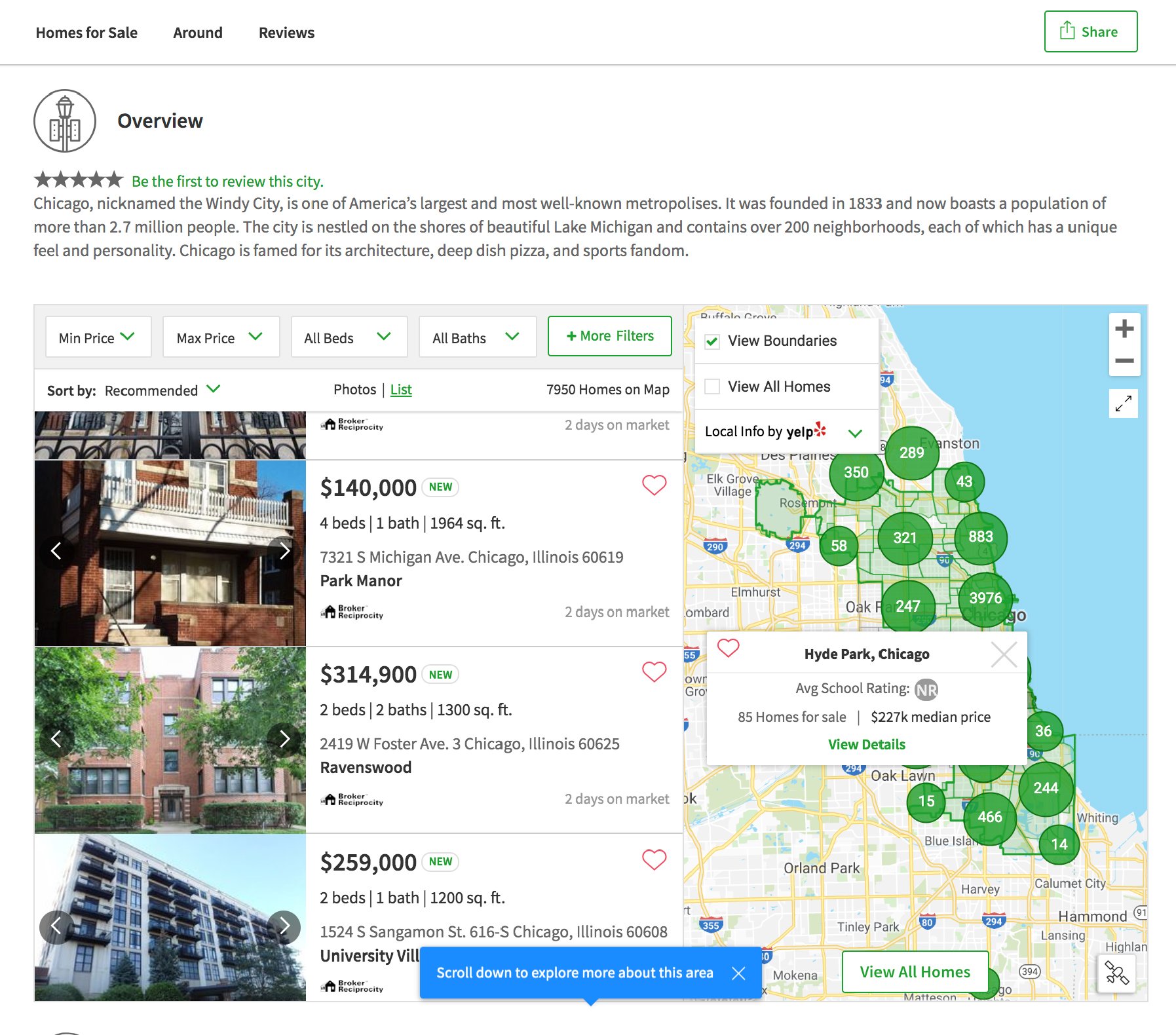### Detailed Descriptive Caption:

This vertical image, accessible via a computer or smart device, features a user interface of a real estate website based on its layout and elements. The interface has a predominantly white background, likely utilizing the white space from the computer screen.

At the top left of the interface, in black text, there are navigational links labeled "Homes for Sale," "Around," and "Reviews." On the top right, there is a green-outlined box labeled "Share" accompanied by a share icon, suggesting options to share the page.

Below these elements, there is a circular icon with the word "Overview" in black text, followed by unfilled stars and a prompt that reads "Be the first to review this city." The section then describes the city of Chicago with an informative blurb stating: "Chicago, nicknamed the Windy City, is one of America's largest and most well-known metropolises. It was founded in 1833 and now boasts a population of more than 2.7 million people. The city is nestled on the shores of beautiful Lake Michigan and contains over 200 neighborhoods, each of which has a unique feel and personality. Chicago is famed for its architecture, deep-dish pizza, and sports fandom."

Further down the interface, there are options to browse homes for sale. On the left-hand side of the image, there are pictures of various houses available on the market. Each listing displays the price, number of bedrooms and bathrooms, square footage, address, neighborhood, and the duration the property has been on the market.

Users can refine their search by setting parameters for the minimum price, maximum price, number of bedrooms, bathrooms, and more filters. On the right-hand side, a map indicates the locations of these homes, visually aiding users in understanding the geographical context of the listings.